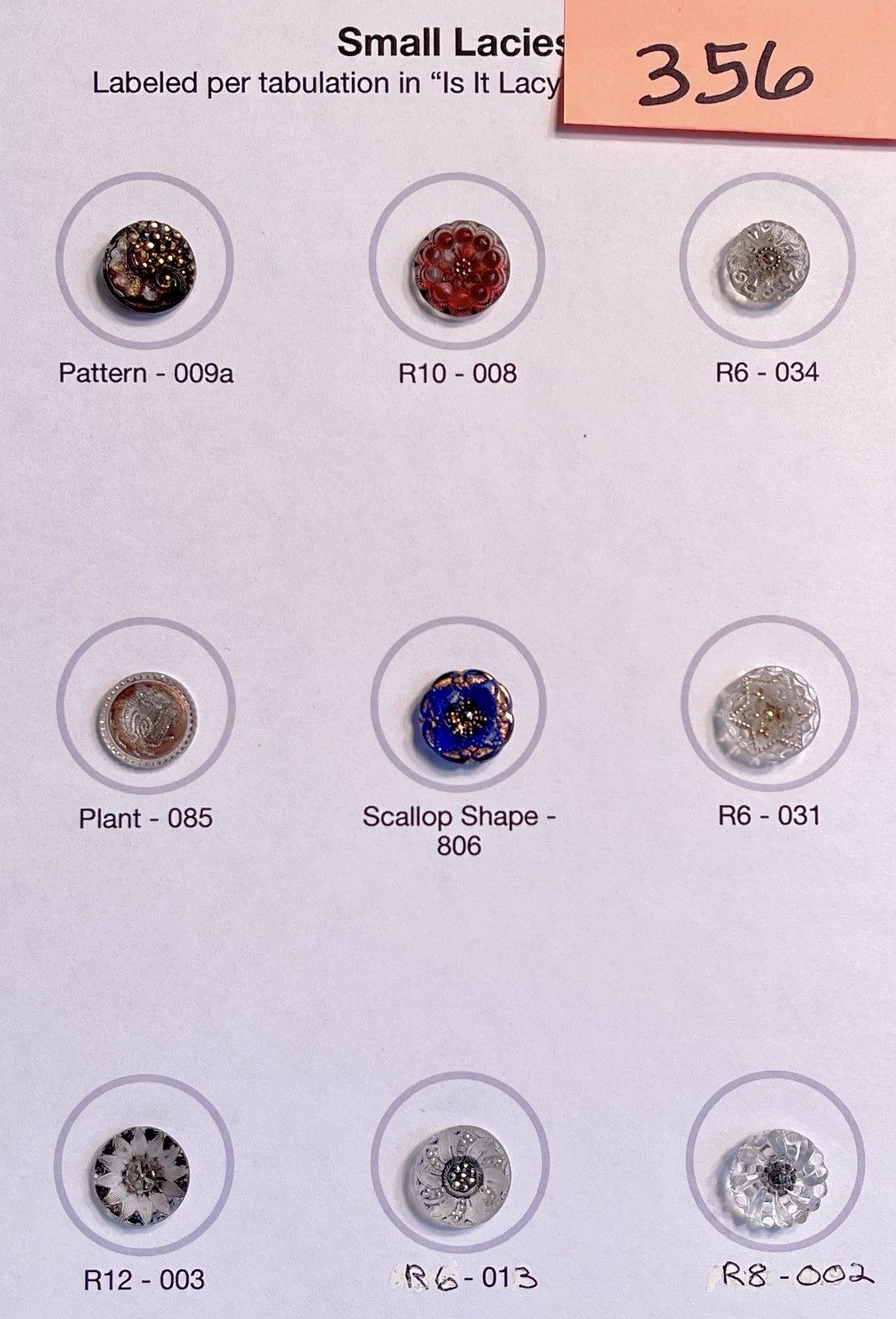The image is a vertical rectangular layout that appears to be designed for sales purposes, showing samples of small laces. The display features nine circular sections, arranged in three rows of three. Each circle contains a unique lace sample, varying in shapes, colors, and patterns, including shades of brown, gray, orange, blue, and some multicolored designs. Above each lace is a black text header reading "Small Laces," and below each lace sample is a label with identifiers such as "pattern-009A," "R10-008," "plant-085," "scallop shape 806," and "R8-002." In the top right corner of the image, there's an orange sticky note with handwritten numbers "356" in black sharpie. Additionally, there is a line of text below the header that reads "label per tabulation," slightly obscured by the sticky note.